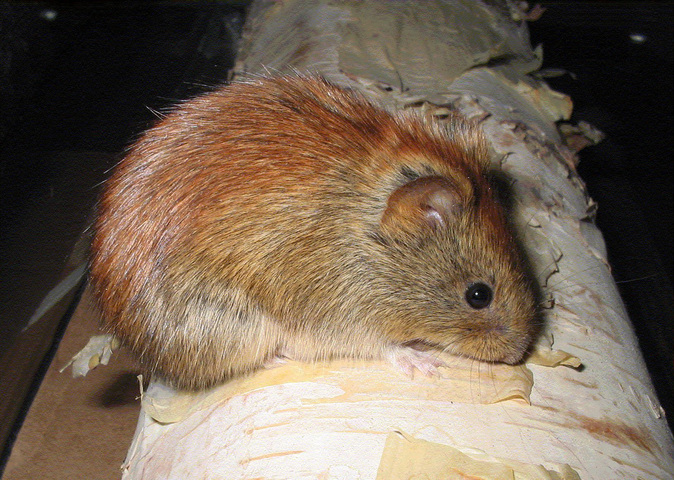This photograph features a close-up of a small rodent, likely a vole, centered prominently within a horizontally oriented landscape frame. The creature, which exhibits a mix of light brown coarse fur that transitions to a reddish hue along its back, is perched atop an old, battered pole wrapped in peeling white tape or cloth. The surface underneath the rodent is scratched and weathered, suggesting extensive wear, and the background is engulfed in deep darkness, accentuated by a light source illuminating the animal from off screen. The vole's right eye, a small black circle, is visible along with one curved ear and a tapered nose, which is pressed downward as though sniffing the surface below. Its face has a grayish tint near the nose, while the right front foot, barely visible, sports three long toes blending into the white surface. Despite the lack of visibility of its tail, the vole's robust hindquarters are notable.